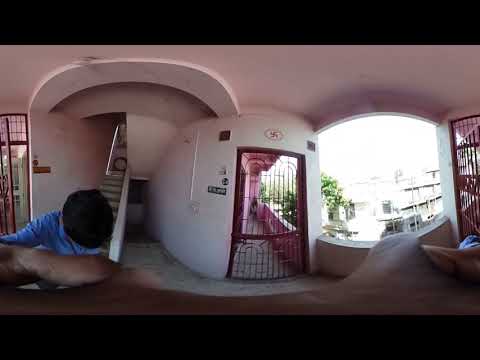The image showcases a fisheye lens perspective from inside an apartment building, capturing the distorted, rounded view of an entry or lobby area. Central to the image is an ornate red metal gate, composed of two archways, set in front of a glass door. On the bottom left, a young boy with black hair, dressed in a blue shirt, can be observed kneeling down, likely holding a smartphone or tablet to take the 360-degree photo, his arms extending outwards and partially visible on both sides of the image. Behind him, a staircase with a rounded arch at the top ascends to the next level.

The building’s interior features light pink stucco walls, adding to its unique architectural charm. To the right of the image, there's a large open balcony space flooded with bright, diffused sunlight, suggesting an overcast atmosphere with evening shadows. Furniture, possibly a couch, is situated in the bottom right corner. The area appears spacious and airy, with a clear view of the cityscape outside. The overall setting hints at a welcoming apartment complex lobby, lined with hallways and housing units.